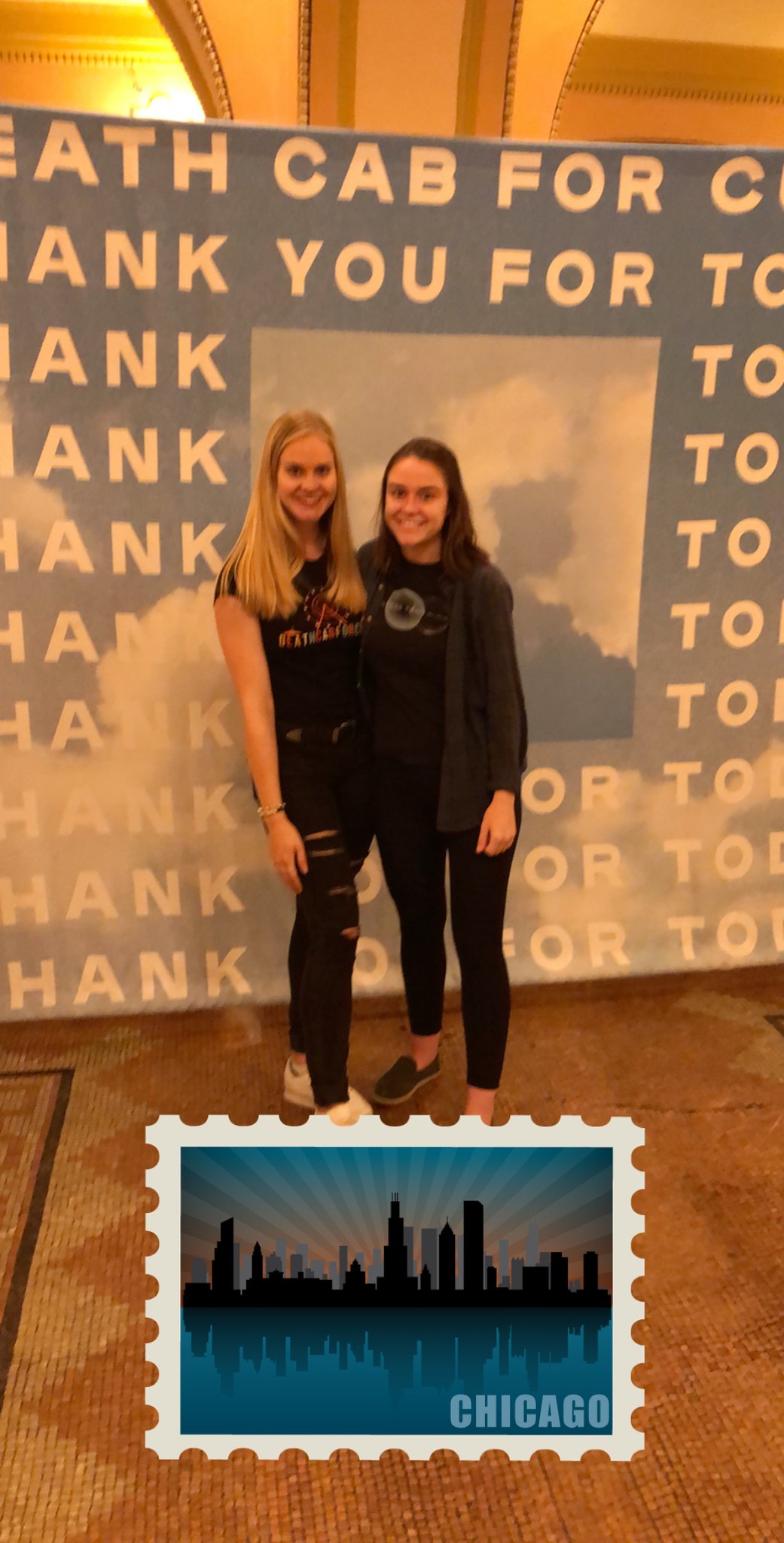The image features two young women, likely in their 20s, smiling and posing together in front of a professionally designed backdrop. The blonde woman on the left is dressed in a black shirt and black ripped jeans, while the brunette woman on the right wears a thin gray coat over a black shirt and black pants or tights. Both women have long hair and display a friendly bond with their arms around each other. The backdrop behind them includes a sky design with partially visible text that seems to advertise an event, possibly related to the band 'Death Cab for Cutie' or a networking event in Chicago. At the bottom of the image, occupying about a quarter of the space and half the width, there's a digital sticker resembling a postcard stamp that highlights the Chicago skyline reflected on a body of water with "Chicago" clearly marked. The setting appears to be an interior space with warm lighting.